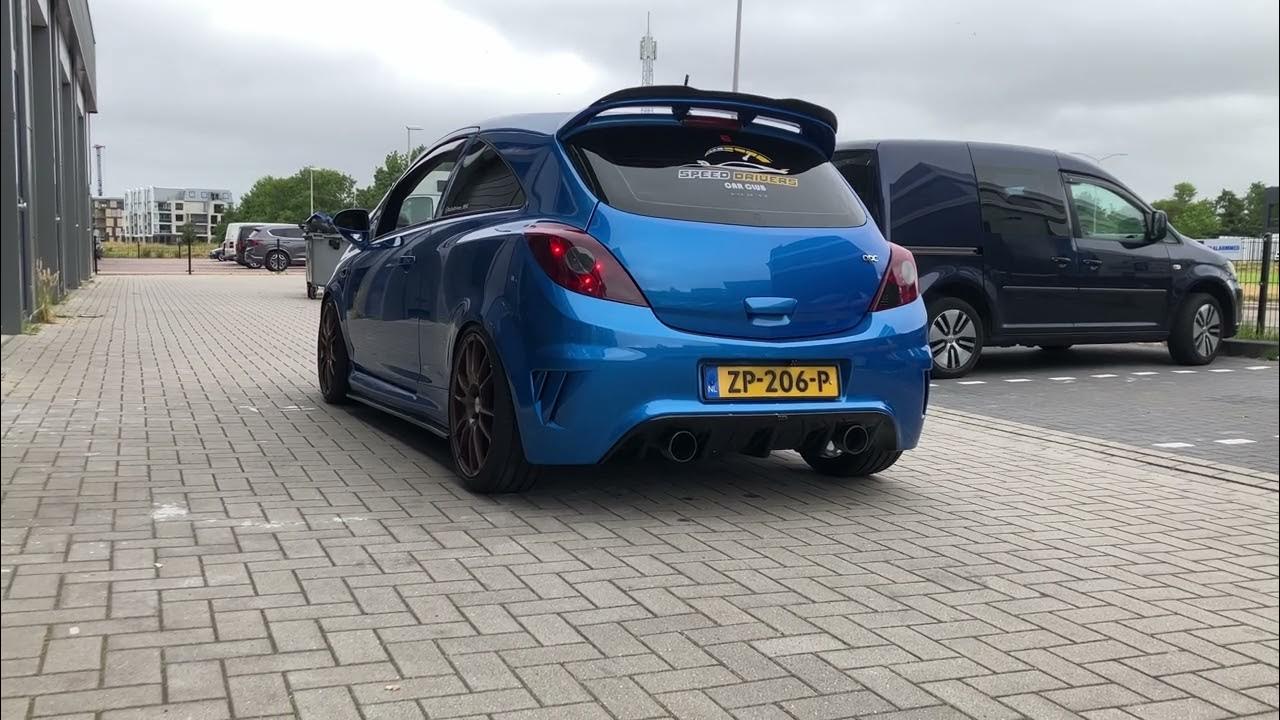The image depicts a cloudy daytime scene in a parking lot, captured in landscape format and in color. The photograph focuses on a shiny, polished blue car with a sporty appearance, including a spoiler and a reflective paint job. The car features a yellow license plate reading "ZP-206P" and has the text "Speed Drivers" along with a logo on the rear window. The car rests on a brick-like patterned surface and appears ready to depart, as it is positioned perpendicular to other vehicles parked diagonally nearby. In the background, there are additional cars and some buildings, all under a sky filled with clouds.